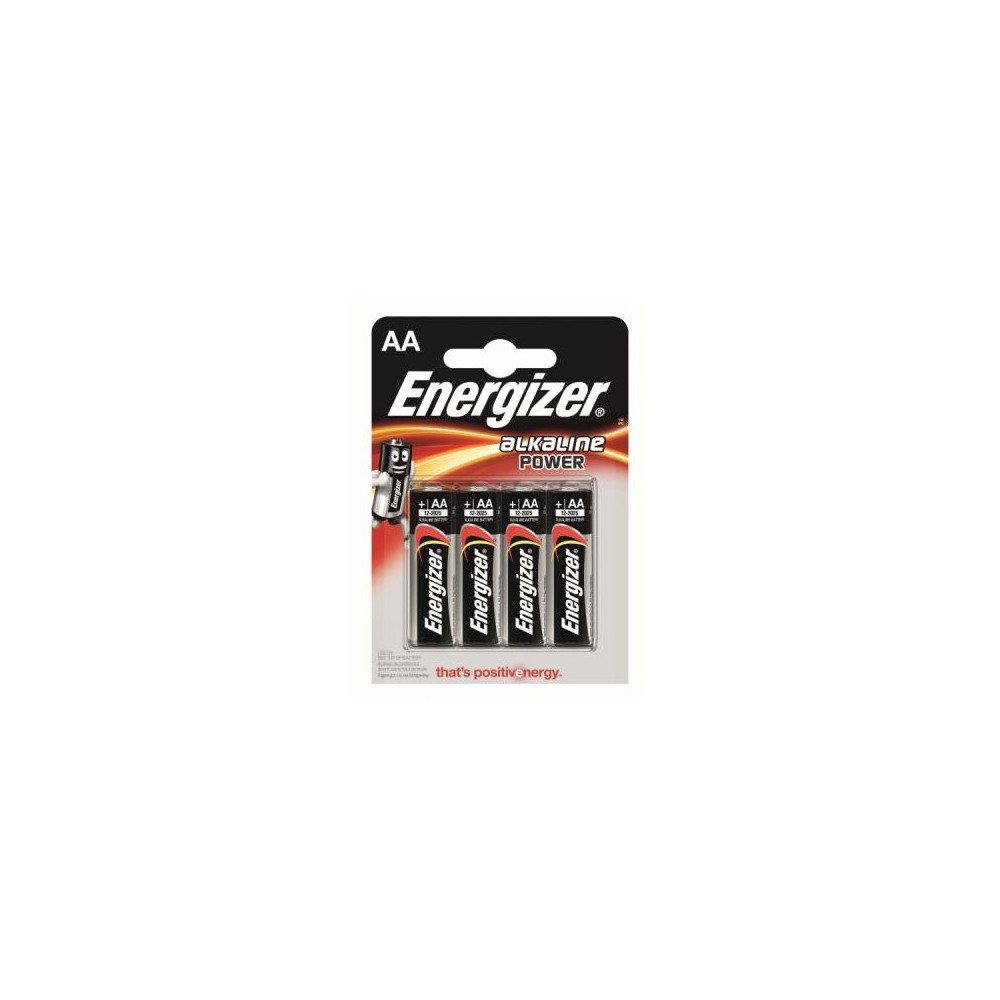This package of Energizer AA batteries is designed for retail display, featuring a hang-tab at the top to easily mount on a store pegboard. The front of the packaging prominently displays the Energizer logo in large white print against a black background. Below the logo, the words "Alkaline Power" are written in white, accompanied by dynamic swishes of red and yellow. 

On the left-hand side of the package, there is a playful illustration of a battery character with arms and legs, appearing to run with a cheerful expression. The character showcases "AA" markings on the front. At the bottom of the package, the phrase "Positive Energy" is prominently displayed.

The packaging includes a clear shrink wrap that houses four AA batteries, allowing them to protrude slightly from the front for easy visibility. The batteries themselves feature a black exterior with red and yellow accents, matching the design elements on the packaging. The remaining background color of the card is a neutral gray, making the vibrant colors and detailed artwork stand out.